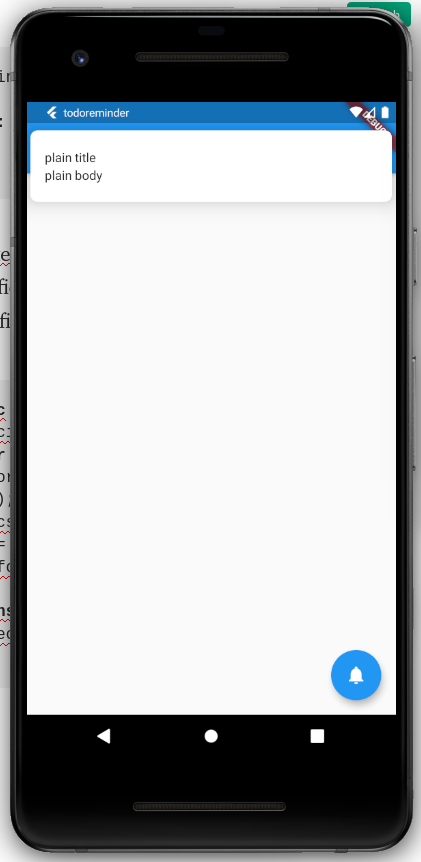This image showcases a black cell phone prominently featuring the To-Do Reminder application. The phone, encased in a sleek black bezel, sports a small forward-facing camera at the top. Below the screen, three navigational buttons are visible: a left arrow, a circle, and a square. 

The app interface, which occupies the screen, is dominated by a large white rectangle designed for note-taking. At the top, within a blue bar, the text "To-Do Reminder" is displayed in white. Directly below this, there is a smaller white box containing gray placeholder text, "Plain Title" and "Plain Body," indicating fields where the user can input the title and body of a note. The majority of the screen is taken up by a large empty space where users can type their notes.

In the bottom right corner of the app interface, a blue circle with a white bell icon is evident, allowing users to set reminders for their tasks. This descriptive setup of the interface makes it easy for users to create and manage their reminders and notes efficiently.